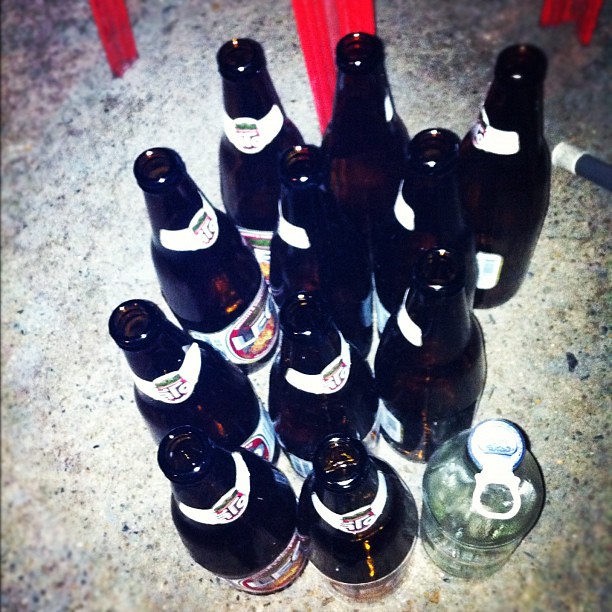The photograph depicts a close-up on a white, speckled concrete floor. The primary focus is on twelve beer bottles arranged on the ground. Eleven of the bottles are made of brown glass, each adorned with white labels around the neck and base, featuring various designs including red logos, the letters "ITO," and other markings that are hard to identify. The twelfth bottle stands out with its clear glass and a silver cap, indicating it likely came in a multi-pack. All the bottles appear to be opened and mostly empty. Surrounding this central scene, at the top of the image, there are faintly visible metallic legs of a stool, while on the top right side, the dark blue end of a plastic chair with a white tip is partially visible. The countertop mentioned appears to be an error, as it is the floor that is described in detail. The photograph seems to be taken with a low-quality camera and a flash, making the speckled floor appear brightly illuminated.